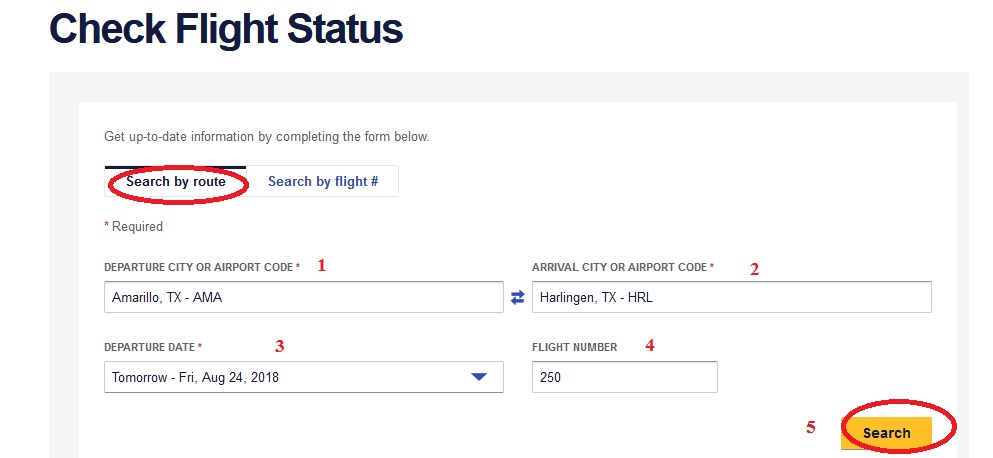This is a detailed caption for the image:

"The image appears to be a screenshot of a flight status checking webpage. At the top left corner, there is a heading that reads 'Check Flight Status.' Below this heading, a subtext instructs users to 'Get up-to-date information by completing the form below.' The form includes two options: 'Search by Route' and 'Search by Flight Number,' with 'Search by Route' circled in red. A note below these options clarifies that fields marked with an asterisk are required.

The first input field is labeled 'Departure City or Airport Code:' followed by suggestions including 'Amaranto, Kansas' and 'Amaranto, Texas.' The next field is 'Arrival City or Airport Code,' with 'Harrington, Texas' filled in. Below this, the form requires the 'Departure Date,' specified as 'Tomorrow, 16 August 2018.' Lastly, there is a field for the 'Flight Number,' which appears to be somewhat illegible but might be '250.'"